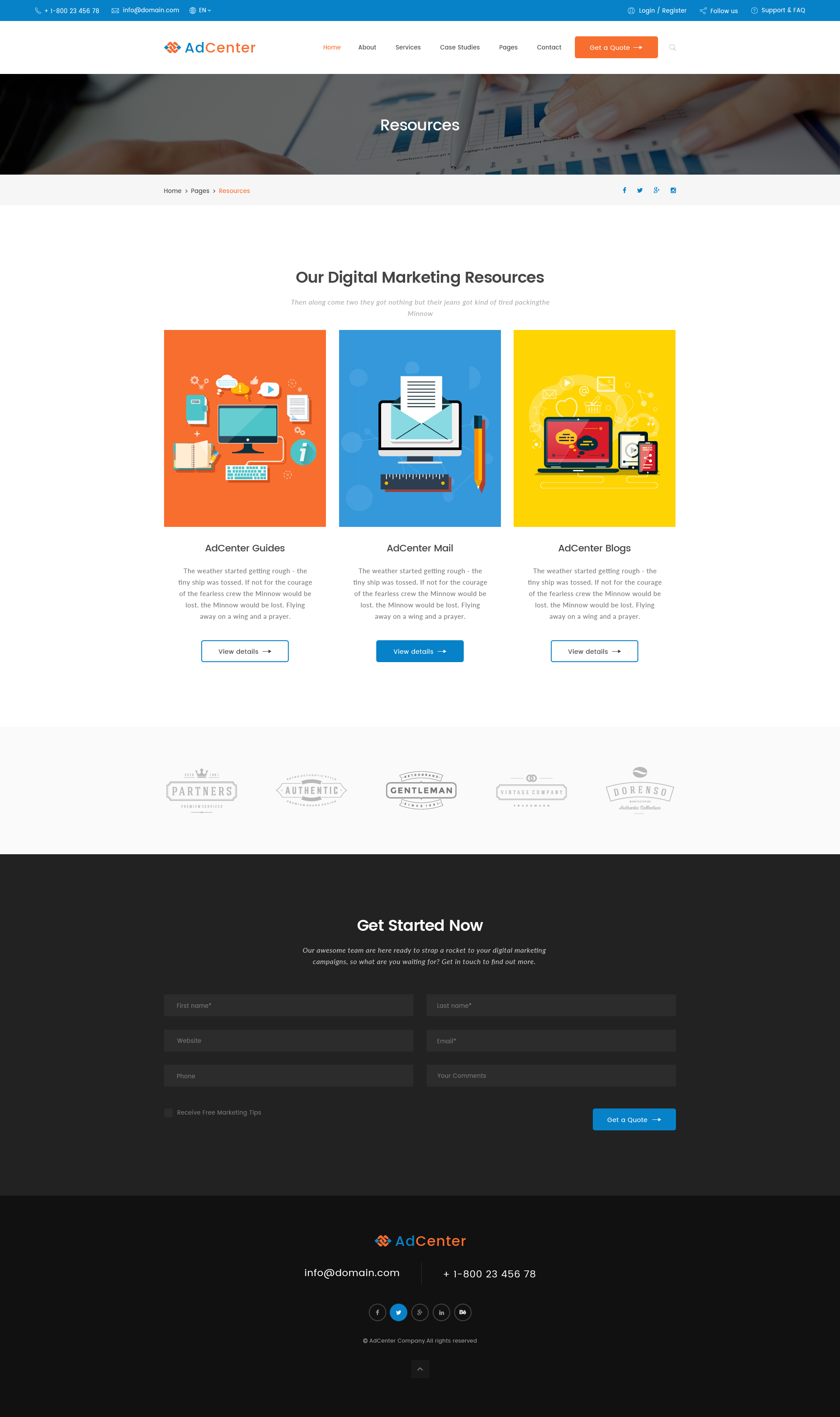### Descriptive Caption

The image depicts a webpage layout with a red header displaying the text "1-800-234-4678" followed by options for "Log In," "Register," "Follow Us," "Ad Center," "Home," "About," "Services," "Case Studies," "Pages," "Contact," and "Get a Quote." Below the header, there is a section labeled "Resources" accompanied by an icon resembling a pen. The navigation menu includes links to "Home," "Pages," "Resources," and social media icons for Facebook, Twitter, and Google. 

The main content area to the left features an orange section with what appears to be a monitor and keyboard illustration, adjacent to an open book and scattered papers. In the center of the image, there is a narrative text about a resilient crew battling rough weather, with repeated phrases for emphasis: "The weather started getting rough, the tiny ship was tossed, if not for the courage of the fearless crew."

Towards the bottom, a call-to-action section encourages visitors to "Get Started Now" or contact the team via the "Contact Page." There’s an enthusiastic note about the awesome team being ready to "strap a rocket to the moon." The contact information is also provided: "info@domain.com" and "1-800-234-567-8."